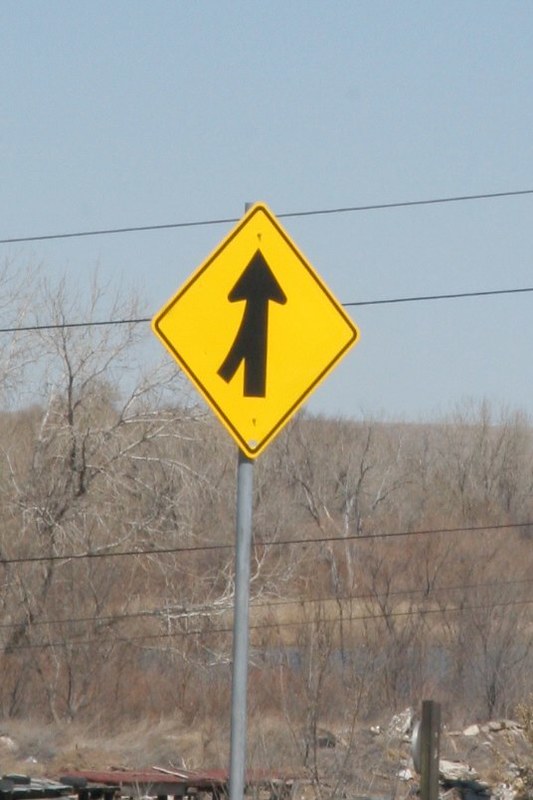A vivid photograph captures a roadside caution sign set against a natural backdrop. The sign is mounted on a sturdy silver metal post and features a diamond-shaped yellow panel bordered in black. Within the yellow panel, a black arrow points upward, merging with an adjacent pathway, indicating that two lanes will combine into one ahead. The background displays a muted grayish-blue sky and a barren landscape, adorned with leafless trees and patches of brown grass, suggesting a late autumn or early winter scene. The entire composition highlights the solitary caution sign amidst the stark beauty of the natural surroundings.